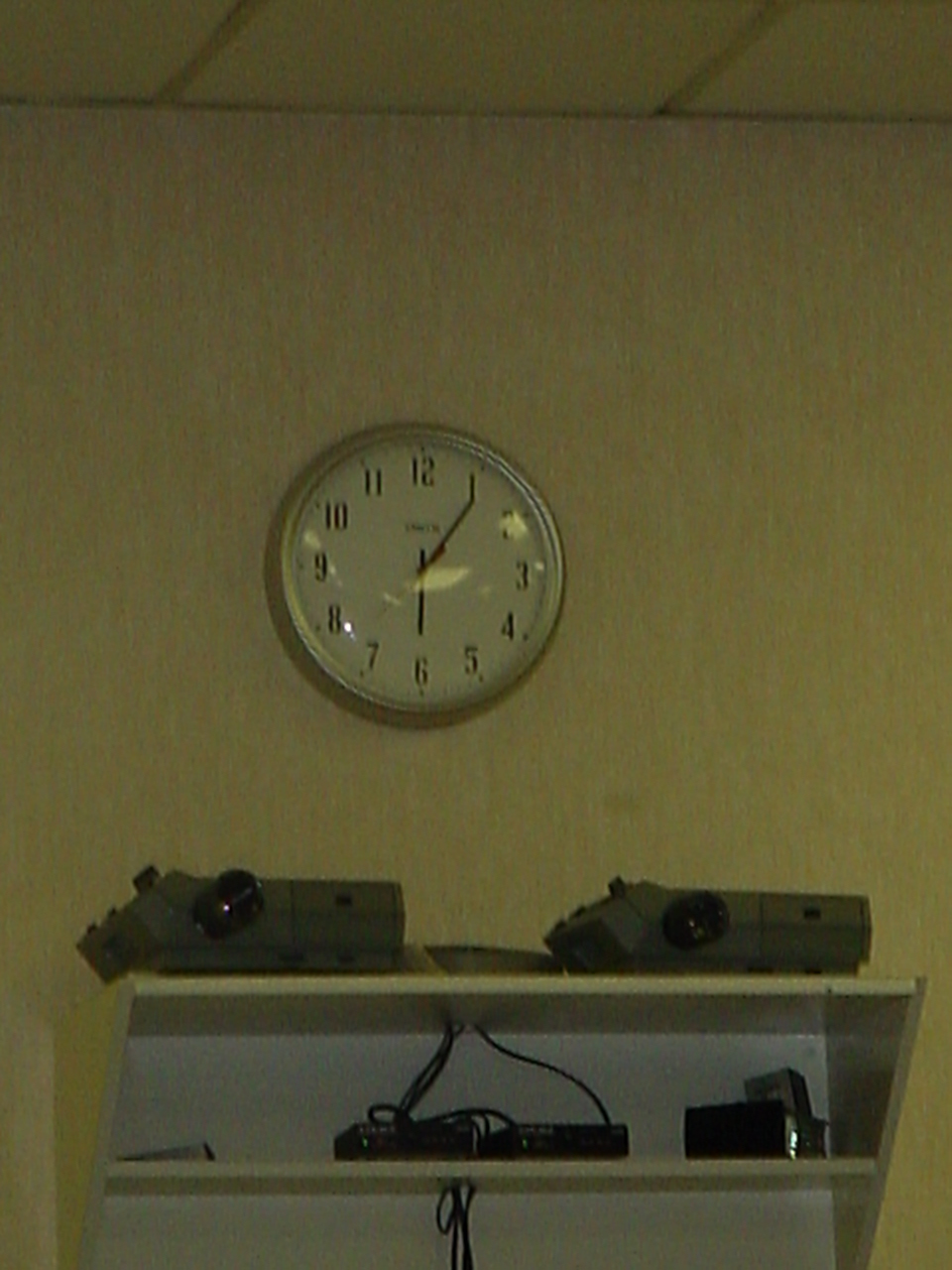This is a slightly blurry photograph depicting a white wall adorned with a round, silver-framed clock. The clock features a white face with black numbers and hands, including a red second hand, and has hash marks encircling the edge of the clock face. Some light reflections are visible on the glass covering the clock. The time displayed is 6:06. Above the clock, a drop ceiling with steel bars is partially visible. Below the clock, a white metal shelf leans against the wall, hosting two silvery-gray projectors with black knobs. Further down, some black electronic devices are connected with visible cords leading up to the projectors. Adjacent to these devices are additional black and silver objects. The entire image has a grainy, textured appearance, emphasizing the slightly yellowish tint of the wall and the meticulous details captured in the scene.